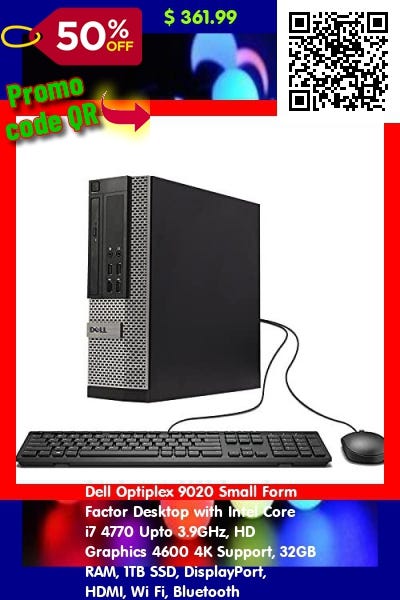The image showcases a promotional QR code for a special offer. In the top left corner of the image, a vibrant red tag displays "50% off" in bold white text. Directly to the right of this tag, the discounted price of $361.99 is prominently shown. Adjacent to the price is the QR code itself, accompanied by the label "Promo Code QR" with an arrow pointing towards the QR code to direct attention.

Below the QR code, there's an image of a sleek black Dell external hard drive tower. It features a grayish front panel, contrasting with the otherwise black exterior. The front panel houses six ports, arranged in two vertical columns of three. Also pictured are a connected mouse and computer keyboard, highlighting the connectivity options available on the back panel.

Beneath the image of the hard drive, descriptive white text specifies the details of the product: "Dell OptiPlex 9020 Small Form Factor Desktop with Intel Core i7-4770, up to 3.9 GHz, HD Graphics 4600, 4K Support, 32 GB RAM, 1 TB SSD, DisplayPort, HDMI, WiFi, and Bluetooth." This comprehensive description emphasizes the high-performance capabilities and modern connectivity features of the desktop, making it an attractive offer at the discounted price.